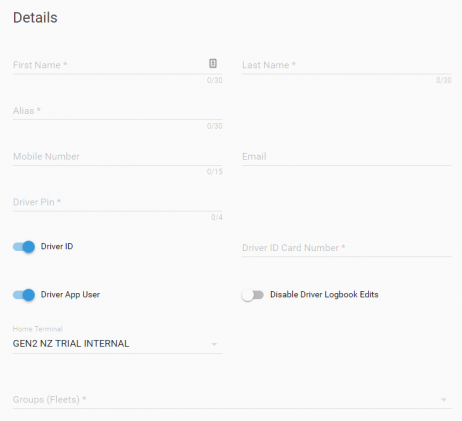The image depicts a grey-themed data capture page with a structured layout and a series of form fields. At the top left corner, in a prominent black font, the word "Details" is displayed. Below this title, there is a series of labeled text boxes and toggle buttons, some of which are not currently editable (opaque).

- **First Line:**
  - On the left: "First Name" with an asterisk.
  - On the right: "Last Name" with an asterisk.

- **Second Line:**
  - On the left: "Alias" with an asterisk.

- **Third Line:**
  - On the left: "Mobile Number."
  - On the right: "Email."

- **Fourth Line:**
  - On the left: "Driver Pin."

None of the above fields are currently editable as they appear opaque.

- **Fifth Line:**
  - On the left: "Driver ID" with a toggle button set to "On."
  - On the right: "Driver ID Card Number," which remains opaque and non-editable.

- **Sixth Line:**
  - On the left: A toggle button for "Driver App User" is set to "On."
  - On the right: A toggle button for "Disable Driver Logbook Edits" is set to "Off."

- **Seventh Line:**
  - On the left: "GEN2NZ TRIAL INTERNAL" in all capital letters.

- **Eighth Line:**
  - On the left: "Groups (Fleets)" with an asterisk, which is also opaque and non-editable.

Each field and button is meticulously organized, yet several fields are currently disabled, indicating restricted access or uneditable states. The use of toggle buttons and asterisks marks mandatory fields and configurable options.